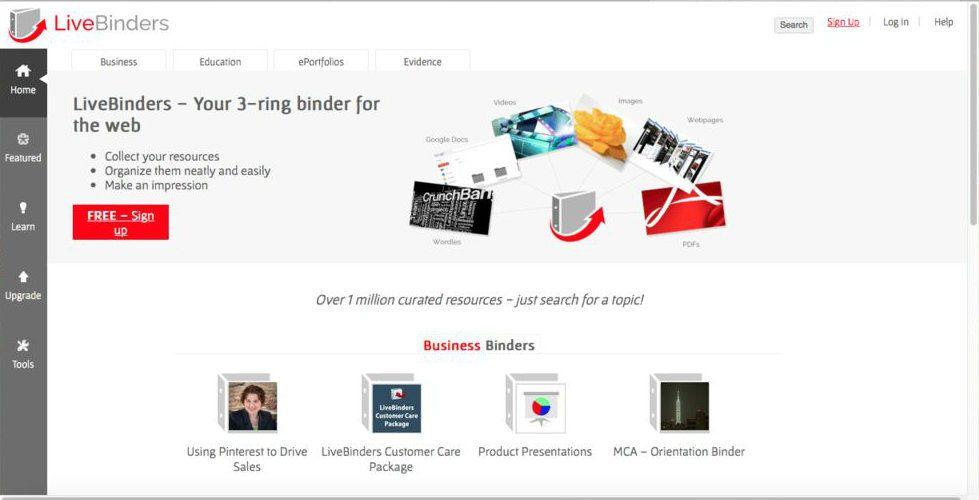A detailed screenshot of a website interface as viewed from a computer or laptop monitor. The website features a predominantly white page layout, with a horizontal gray navigation bar at the top and a vertical gray sidebar on the left. 

In the upper left corner of the website, there is a notebook icon accompanied by a red arrow that swoops up to the right, with the red text "LIVE" to the right of the arrowhead. Further to the right, there is the word "BINDERS." On the far right of the top navigation bar, there is a rectangular gray button labeled "Search" in black text, beside an illegible red text element. Adjacent to the search bar, there are "Log In" and "Help" options in black text. The far edge of the page features a dark gray scroll bar.

Directly beneath the top navigation bar, a secondary gray section includes four black-labeled tabs: "Business," "Education," "e-Portfolios," and "Evidence." Below these tabs, the bolded text "Live Binders, your three-ring binder for the web" appears prominently. 

The central content of the page is structured with three bullet-pointed sentences beneath the primary heading. Toward the bottom left of the page, a rectangular red button with white lettering says "Free Sign-up." 

On the right-hand side of the page, a roughly circular image displays various screenshots of websites labeled with "Google Docs," "Videos," "Images," "Webpages," "PDFs," and what appears to be "Word Files" or "Word Lists." The same binder icon with the red arrow from the top left corner appears again at the center of this section.

At the bottom of the page, there's a statement in black text noting "Over one million curated resources, just search for a topic," followed by the words "Business" in red and "Binders" in gray. Below this, three notebook icons are presented, each with a corresponding title.

The vertical gray sidebar on the left-hand side of the page includes several white icons with accompanying labels: a home icon labeled "Home," a star labeled "Featured," a light bulb labeled "Learn," an up arrow labeled "Upgrade," and a wrench labeled "Tools."